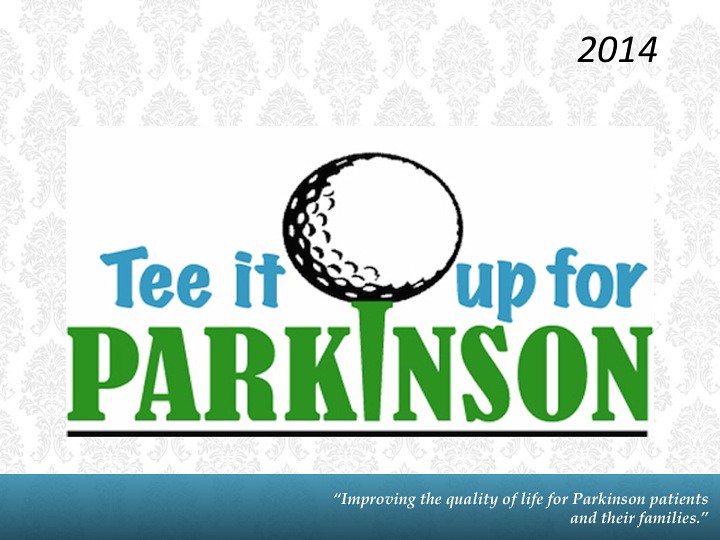In the image, we see a white background with a centrally located logo. The logo features a white and black sketch of a golf ball with visible dimples at the top of the letter "I", resembling a tee. Below the ball, the phrase "T It Up For" is written in light blue text, followed by the word "Parkinson" in grass-green text. The logo text forms "T It Up For Parkinson," with the "I" ingeniously designed to look like a golf tee supporting the ball. A thin black line appears beneath the word "Parkinson." In the upper right corner of the image, the year "2014" is inscribed in black text. The footer of the image contains a light blue rectangle with the slogan "Improving the quality of life for Parkinson's patients and their families" written in white. The background includes a subtle, repetitive floral or leaf pattern in light black, adding an elegant touch.